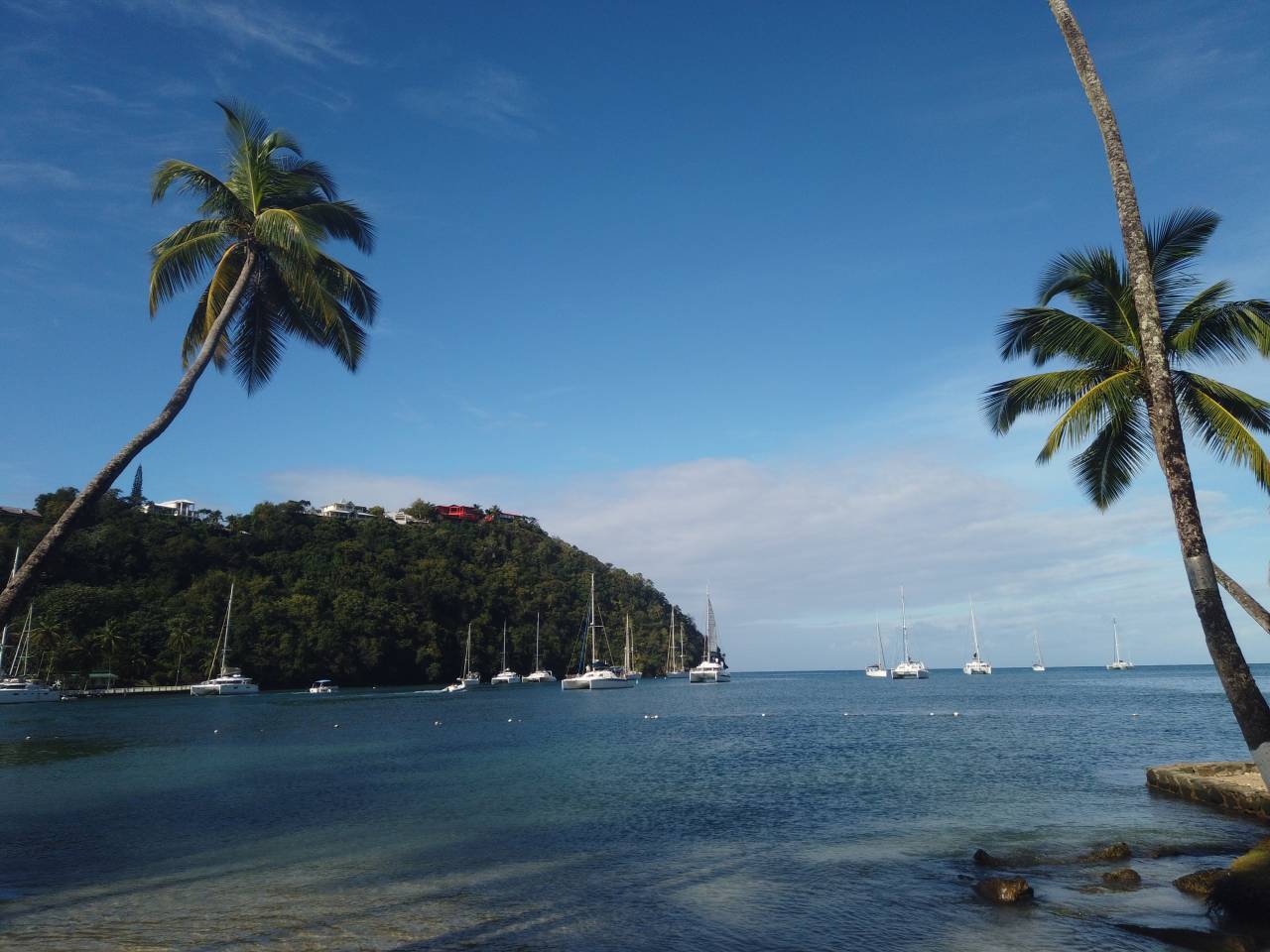This captivating image showcases a picturesque coastal scene, likely a beach or harbor. The photo features two prominent palm trees framing the composition, one on the far left and the other on the right side of the image. The majority of the view in front is serene, expansive water, stretching across the bottom quarter of the vertical plane, punctuated by several white sailboats and yachts scattered across the waves, possibly numbering up to fifteen. 

In the mid-ground, the water meets a grassy mountainside that rises towards a hilltop adorned with a cluster of homes, visible as white and red specks among the greenery. A small section of beach is hinted at but mostly obscured by rocks and possibly some cement structures on the right side of the photo. 

Above the tranquil sea, the sky is beautifully clear, with a vivid blue expanse dominating the upper portion, accented by wisps of cloud cover near the horizon, some with a slight purplish hue. The overall scene captures a vibrant, sunny day, evoking the warmth and natural beauty of a tropical coastal environment.